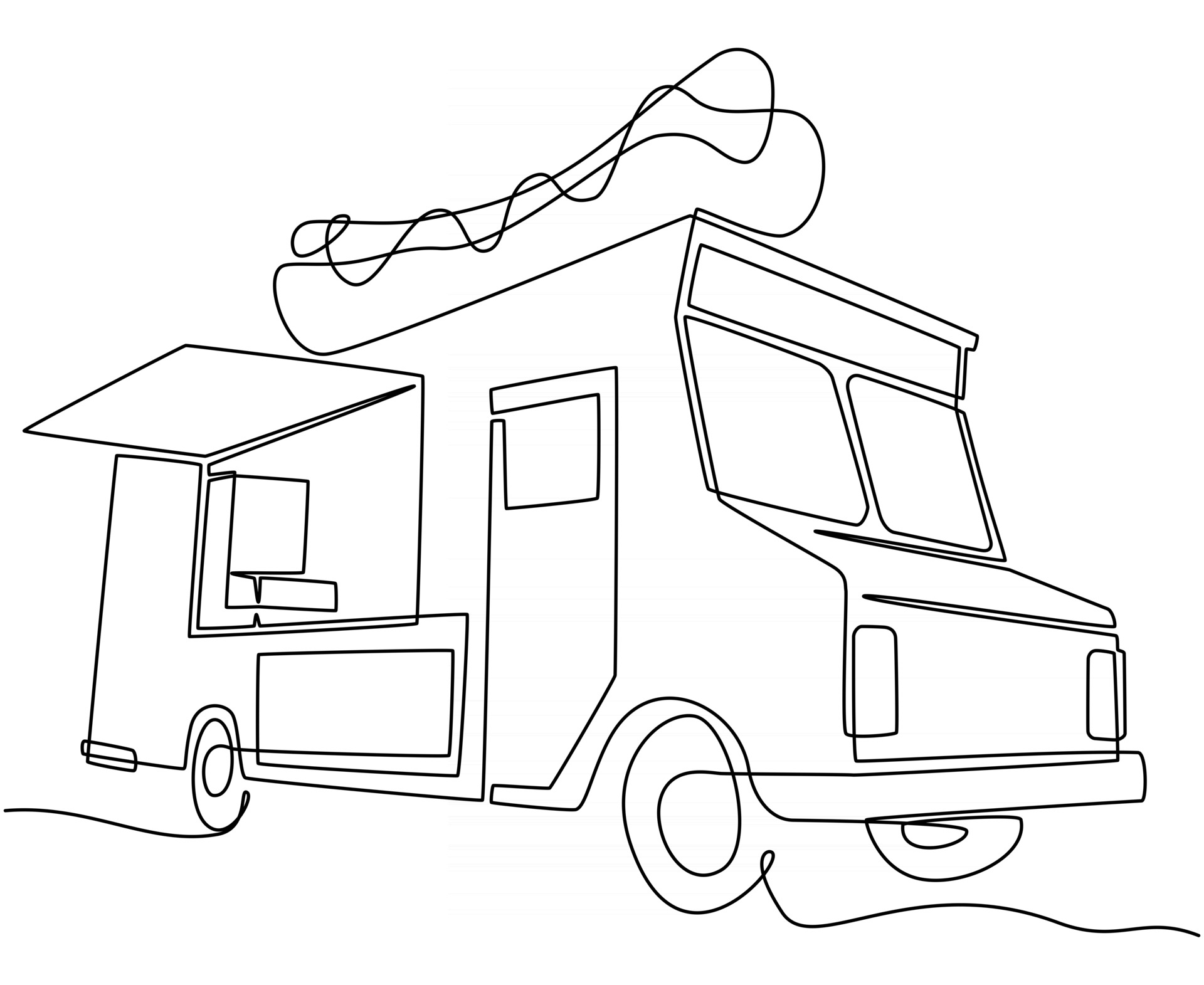The image showcases a digitally drawn, black-and-white lineart illustration of a food truck, created using a continuous single line. The thick black line begins on the left and skillfully traces the outline of the truck, forming the wheels, body, and door in one unbroken motion. Atop the food truck is a large, crudely shaped hot dog, presumably serving as its logo. The truck's side flap, reminiscent of ice cream trucks, is open, but no interior details such as a cash register or customers are visible through the windows. The truck faces right and stands out against a plain, detail-less background.